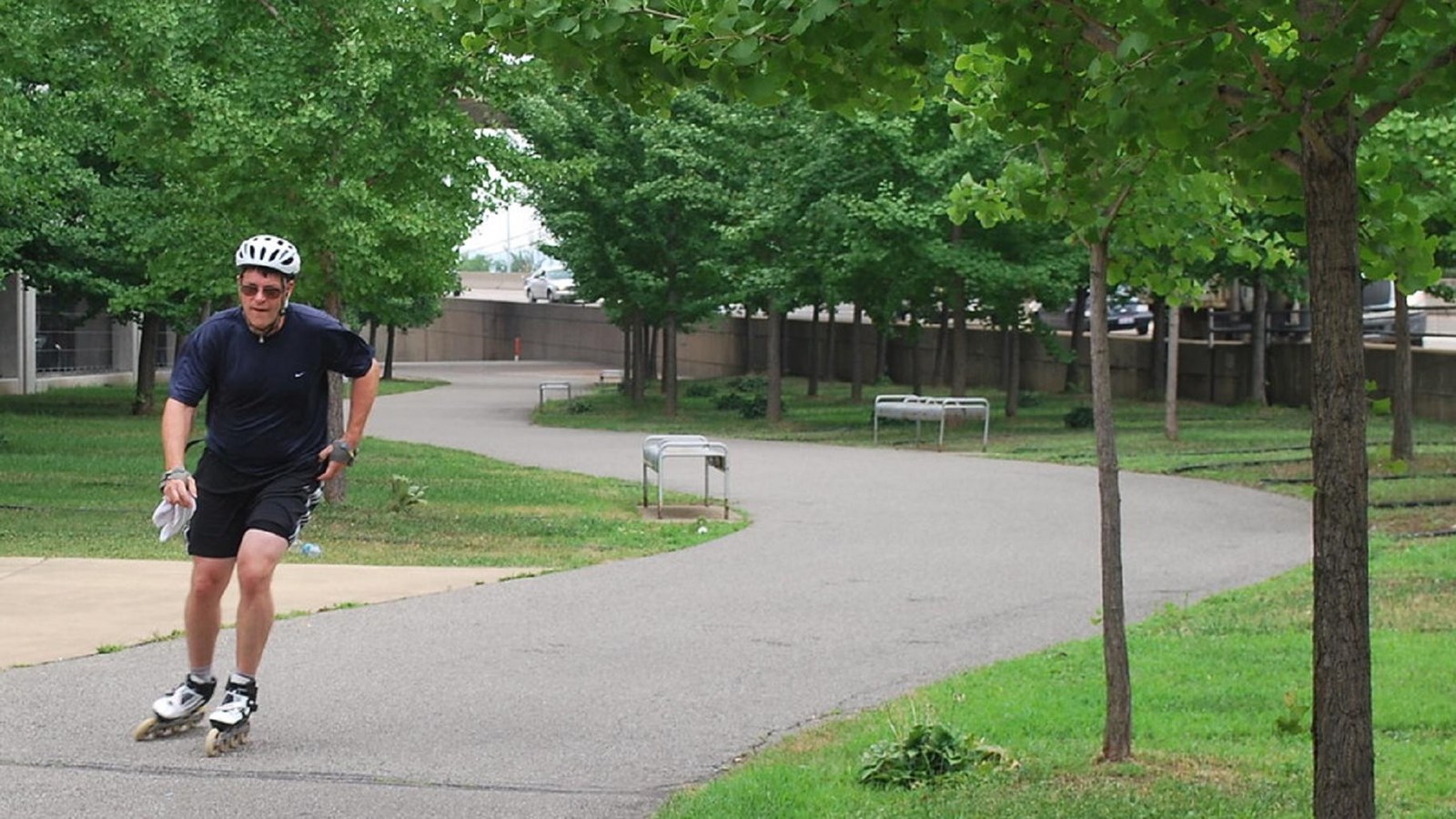The image captures a man rollerblading in a park on a warm day. Positioned towards the left side, he is equipped with a white helmet, prescription sunglasses that appear dark, a black Nike shirt, and athletic shorts, complemented by white and black rollerblades. His hands are wrapped with protective gear, suggesting he is an experienced skater. The park features a winding asphalt trail that zigzags through lush greenery, including many trees and occasional bushes. In the distance, you can see a parking lot and a small hill. The park also has benches and appears to be well-maintained, with trees still full of leaves. The scene is serene with no other people in the background, emphasizing the man's solitary enjoyment of the park's amenities.